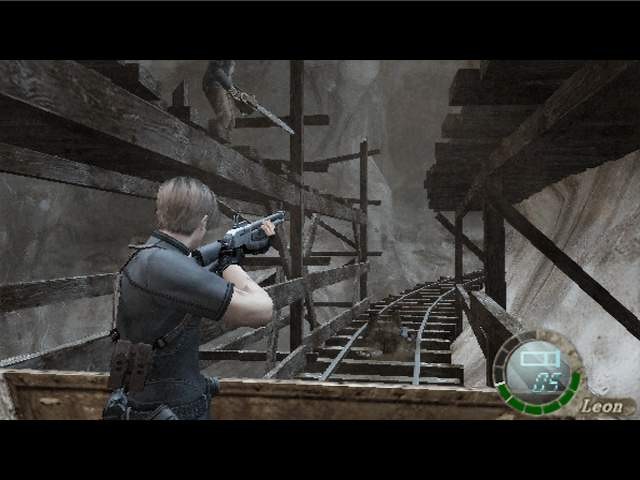The image is a still from a video game, likely resembling a first-person shooter such as Call of Duty. On the right side of the screen, a score indicator is visible, displaying the number 5 inside a circle. This circle is partially lit in green, with some segments grayed out, which likely indicates the number of kills or objectives remaining in the game.

In the foreground, there is a young man with medium brown hair, dressed in a black shirt and wielding a black machine gun. He appears to have a holster or some equipment strapped to his back. He is shown firing his weapon, presumably at an opponent or target.

In the background, another character is positioned slightly higher on the screen and is also armed. They are situated on a platform made of elevated wooden pieces. The scene is set within a tunnel, featuring a train track running down the center, adding to the dynamic and intense atmosphere of the gameplay.